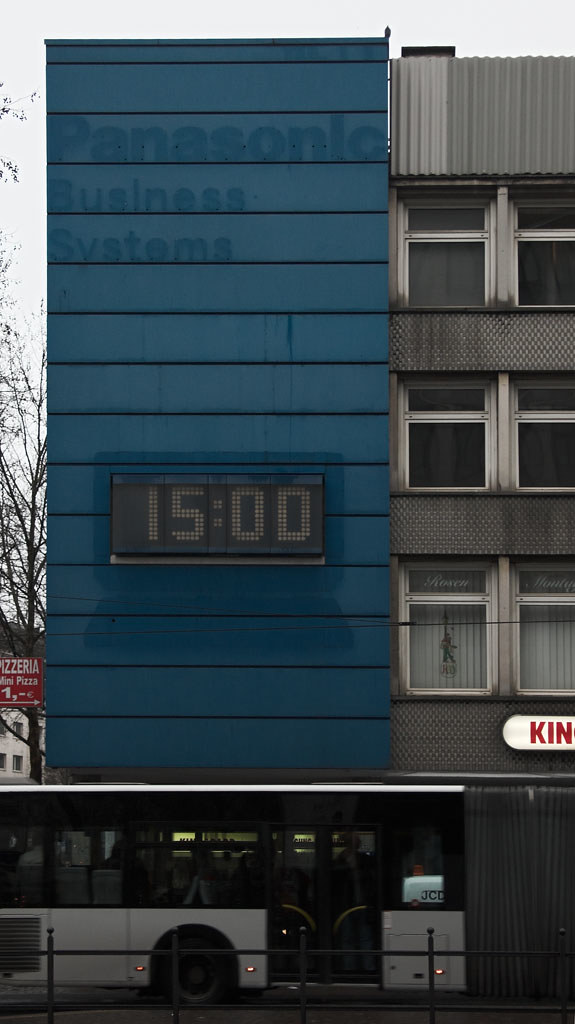In this image, we see a detailed urban scene featuring a section of a building and a local city bus. The lower part of the image displays a gray railing composed of one horizontal line and five vertical pickets. Behind the railing is the back end of a city bus characterized by a light gray lower section, black tires, and an upper part that is mostly black with a top white line, complemented by large windows.

To the right of the bus, the lower part of the building is gray, above which is a partially visible sign reading "KIN" in red text against a white background. The left side of the building is highlighted in blue with the word "Panasonic" prominently displayed, followed by "Business Systems" also in blue text. Below this signage, a rectangular digital clock displays the time as "15:00".

The right-hand side of the building is gray and features six windows evenly spaced across its surface. This detailed composition showcases the intersection of public transportation and urban infrastructure.